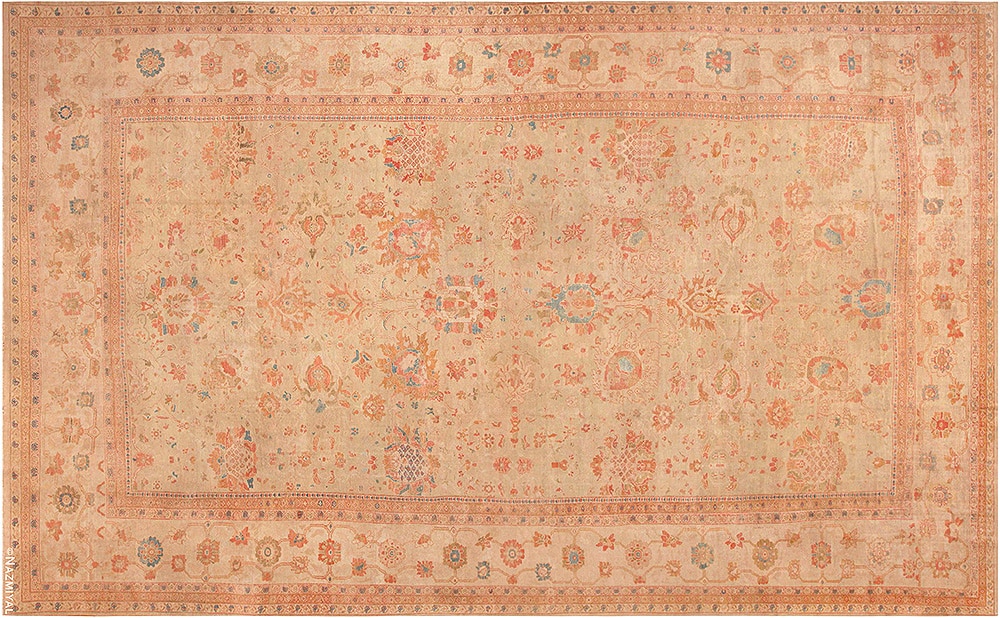This image captures an overhead view of a very old, worn brown rug. The rug is rectangular in shape and features a thick border adorned with an ornate pattern. Inside the border, there is an additional rectangular section decorated with an interlocking floral pattern. Enclosed within this section is yet another rectangle, mirroring the outer pattern. The innermost rectangle displays a broad area of large, stylized floral prints. The entire design is significantly faded, exhibiting a predominantly brown tone with hints of blue and purple scattered throughout. In the lower left corner, a copyright symbol and the sideways text "NAZMIYAL" are printed in white letters.